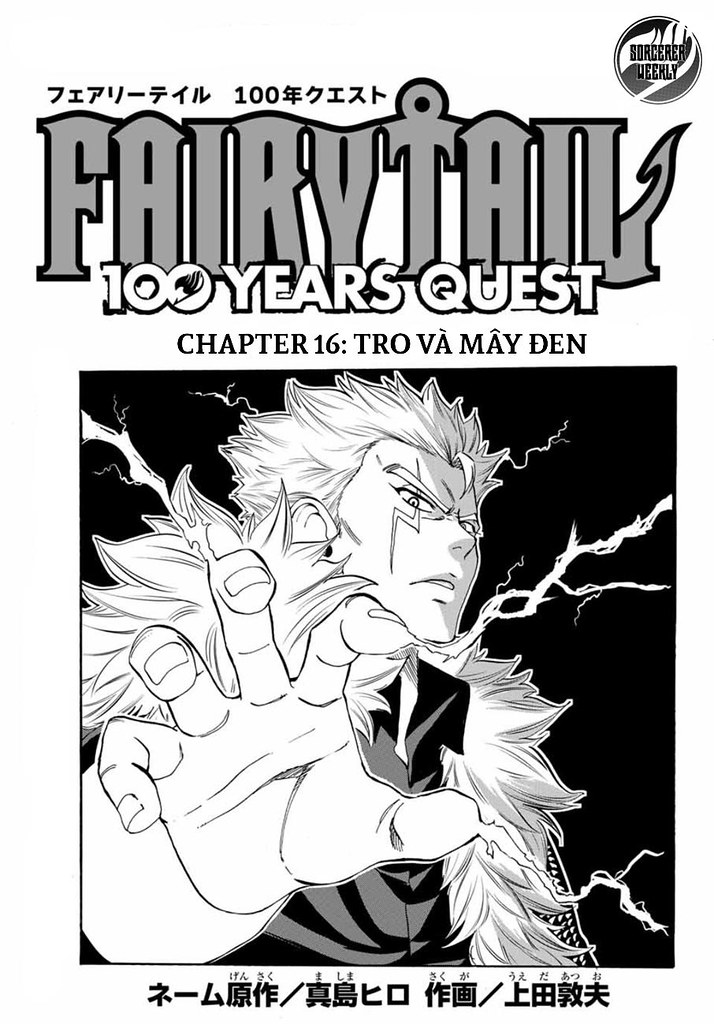This black and white scan of a manga cover features Chapter 16 of "Fairytale 100 Years Quest" titled "Trova Meiden." The top of the page includes the series logo with some Japanese text above "Fairytale" and more Japanese text at the bottom. A prominent circular symbol in the top right corner reads "Sorcerer Weekly." Central to the image is a detailed drawing of a character with spiky, swept-back hair, looking menacingly downward. The character, sporting a distinctive lightning bolt-shaped scar beneath their left eye, reaches out towards the viewer with their hand, from which electricity dramatically shoots out, extending from their fingertips and thumb. Additional lightning emerges from their body and hair, set against a stark black background, enhancing the dynamic and electrifying atmosphere.